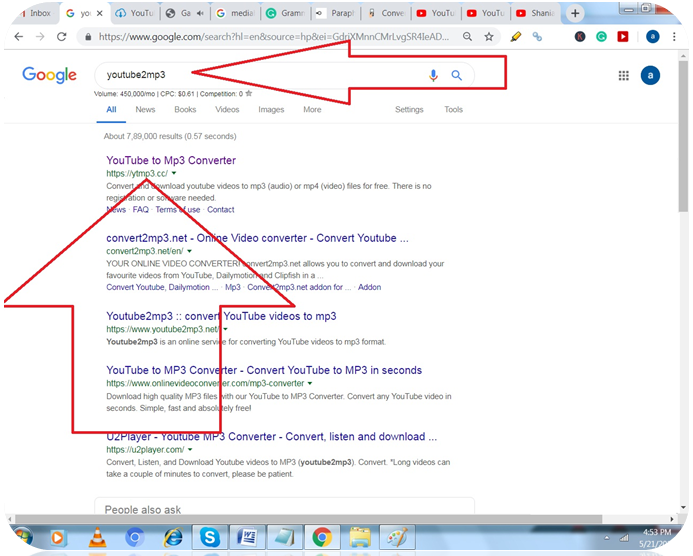In this detailed screenshot, the upper left corner displays several minimized tabs, including "Inbox," "YouTube," "Google Media," and "Grammarly." Two additional "YouTube" tabs are also visible. The address bar shows the Google search page with the URL "www.google.com/search." The primary search bar contains the query "YouTube to mp3," highlighted by an edited red arrow. Below the search bar, a list of search results is visible, with another red arrow pointing to the top result titled "YouTube to MP3 converter." Subsequent results include links such as "convert2mp3.net," "YouTube to mp3," and another "YouTube to MP3 converter."